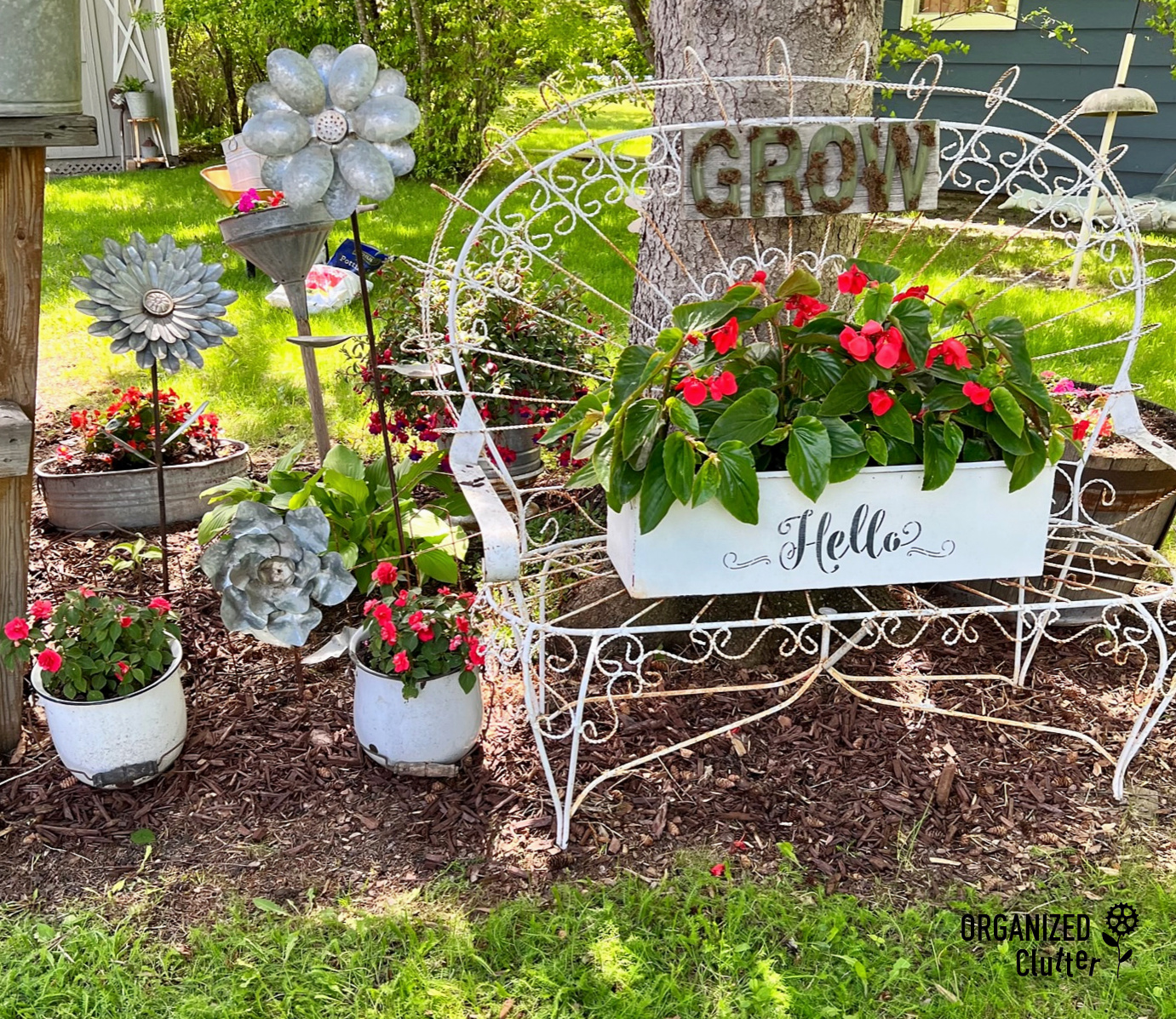The image features a vibrant garden scene with a central focus on a white, rust-speckled metal bench adorned with intricate wavy designs. Located in front of a tall tree trunk, the bench has a decorative sign that reads "grow" at the top. Placed on the bench is a white planter box with the word "hello" displayed in black lettering, filled with red flowers and shiny green leaves. The area beneath the bench is covered with dark brown wood chips, contrasting with the lush green grass that spreads across the garden. To the left of the bench, two white flower pots contain pinkish-red flowers and greenery. Additionally, garden embellishments like metal flower-shaped decorations on stakes enhance the left side of the scene. The background features a bright green lawn with some sunspots, a tree trunk, and a partial view of a house with blue wooden siding in the upper right corner. The garden is filled with happy colors of green and yellow, creating a cheerful and inviting atmosphere.